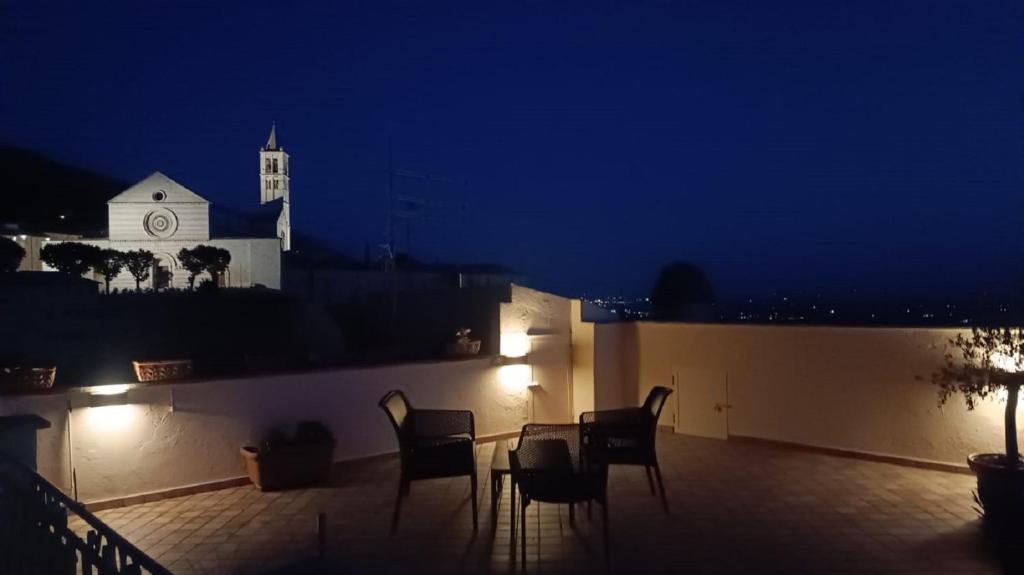Captured at night, the photograph presents a serene outdoor recreational area, likely a private terrace or veranda in a residential setting. The dark blue, almost black sky sets a dramatic backdrop, while subtle lighting shapes the scene. Three unseen lights provide a gentle glow, illuminating the main focus—a small table surrounded by three outdoor chairs at the center of the image. Enclosed by waist-high walls of white adobe and a section of wrought iron fence, the space feels intimate yet airy. 

Along the edges, details emerge: a small hatch door on one side, several baskets on another wall, and a rectangular pot with a plant on the leftmost wall. Also noticeable is a separate pot on the right side, housing a small tree. Closer to the observer, there is a gated entrance shrouded in darkness, its color and material indeterminate. In the distance, a lit white building with a distinct two-tiered structure and a prominent church or steeple stand out against the night sky. Farther away, a tower with an indistinguishable flag hints at a broader urban landscape, completing this picturesque nocturnal scene.